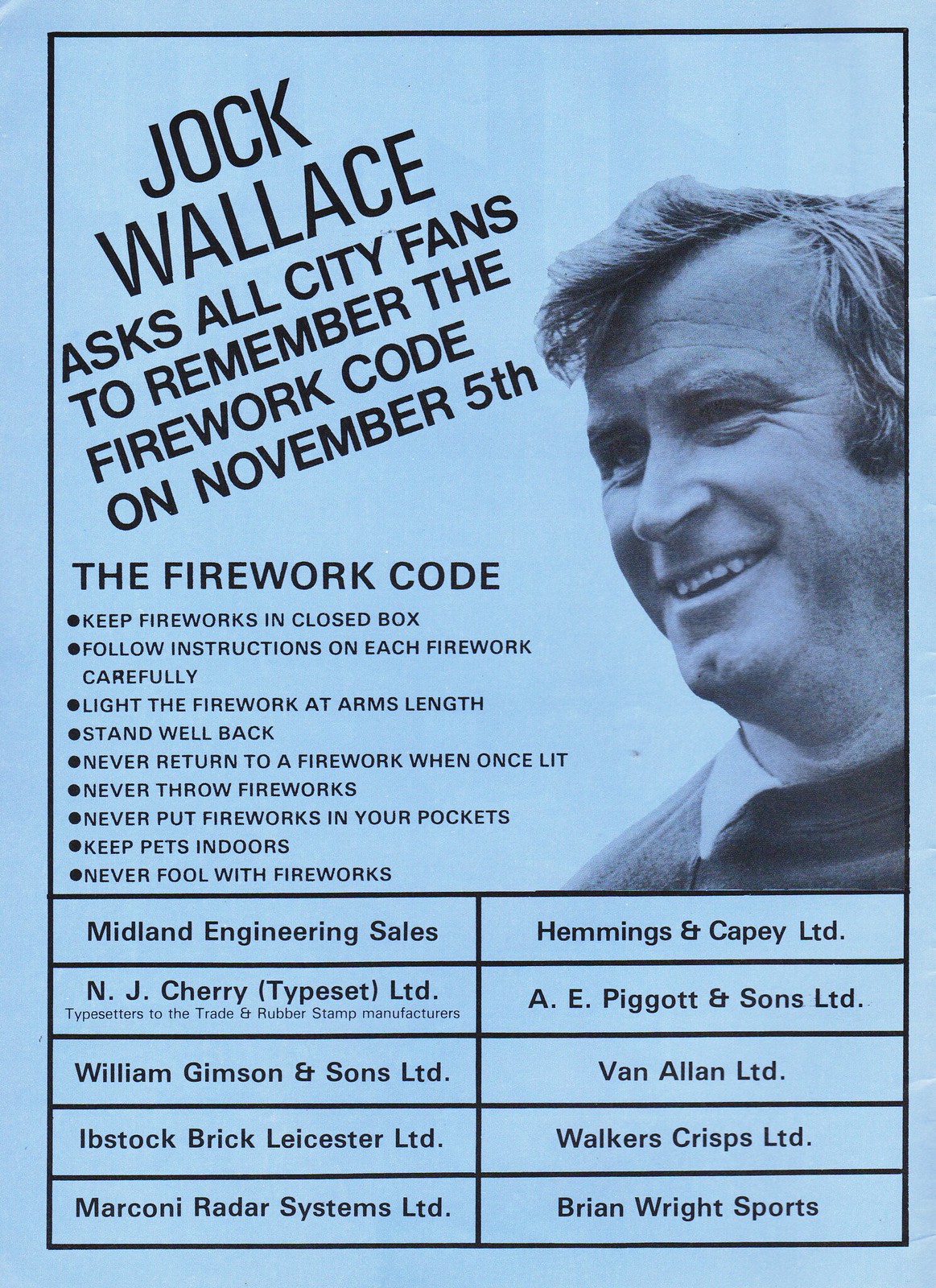The poster, set against a light blue background with black accents, is a public service announcement by Jock Wallace urging all city fans to remember the firework code for November 5th. The top of the poster features a prominent black-bordered box containing a tilted black font header: "Jock Wallace asks all city fans to remember the firework code on November 5th." Below this, in straightforward font, the firework code is outlined in detailed bullet points: 
- Keep fireworks in a closed box.
- Follow instructions on each firework carefully.
- Light the firework at arm's length.
- Stand well back.
- Never return to a firework once lit.
- Never throw fireworks.
- Never put fireworks in your pockets.
- Keep pets indoors.
- Never fool with fireworks.

On the right side of the poster is a black-and-white image of a man, presumably Jock Wallace, smiling with a distinctive dimple in his chin to add a personal touch to the safety message. Below the firework code, a series of ten rectangular boxes list various companies supporting the announcement. In the left column: Midland Engineering Sales, NJ Cherry Typeset, William Gibson and Sons, Hipstock Brick Leicester, and Marconi Radar Systems. In the right column: Hemmings and Cappy, A.E. Peegle and Sons, Van Allen, Walker Crisps, and Brian Wright Sports. The announcement effectively combines a strong visual element with the critical text, highlighting the importance of firework safety and community support.